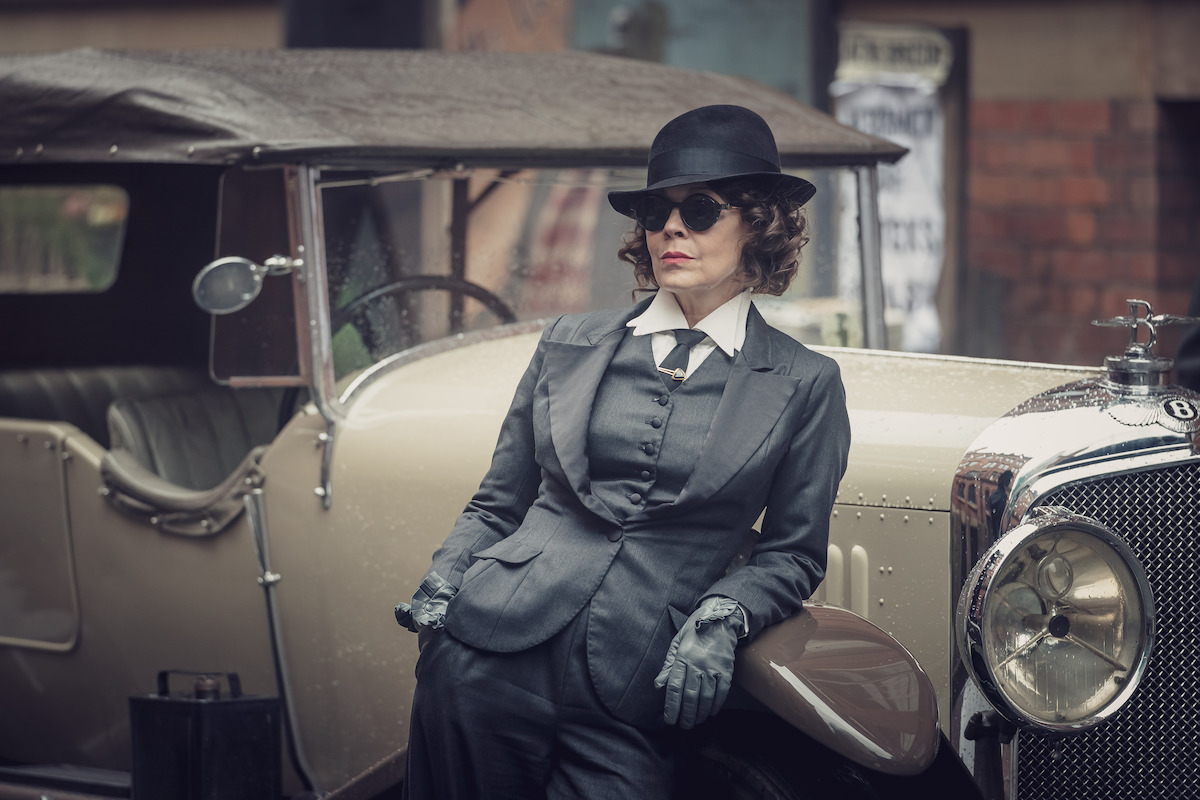In an evocative scene reminiscent of the TV series Peaky Blinders, a poised woman stands centered in the image, exuding vintage elegance. She wears a tailored three-piece gray suit over a crisp white, double-collared shirt, accented by a gray tie with a diamond tie clip. Her look is completed with light gray gloves, a stylish hat, sunglasses, curly hair, and striking red lipstick. She leans nonchalantly against a meticulously restored classic car, likely a Bentley from the 1930s, with a gleaming silver chassis and a distinctive, screen-like front grill. The car occupies the majority of the image, with its hood visible at the bottom right and the passenger section extending to the far left. Behind the car, a brick wall is exposed, particularly in the upper right corner, adding to the vintage ambiance with its rustic texture. There's no text in the image, allowing the array of colors—black, white, a hint of red, silver, tan, and brown—to convey the elegance and historical charm of the era.